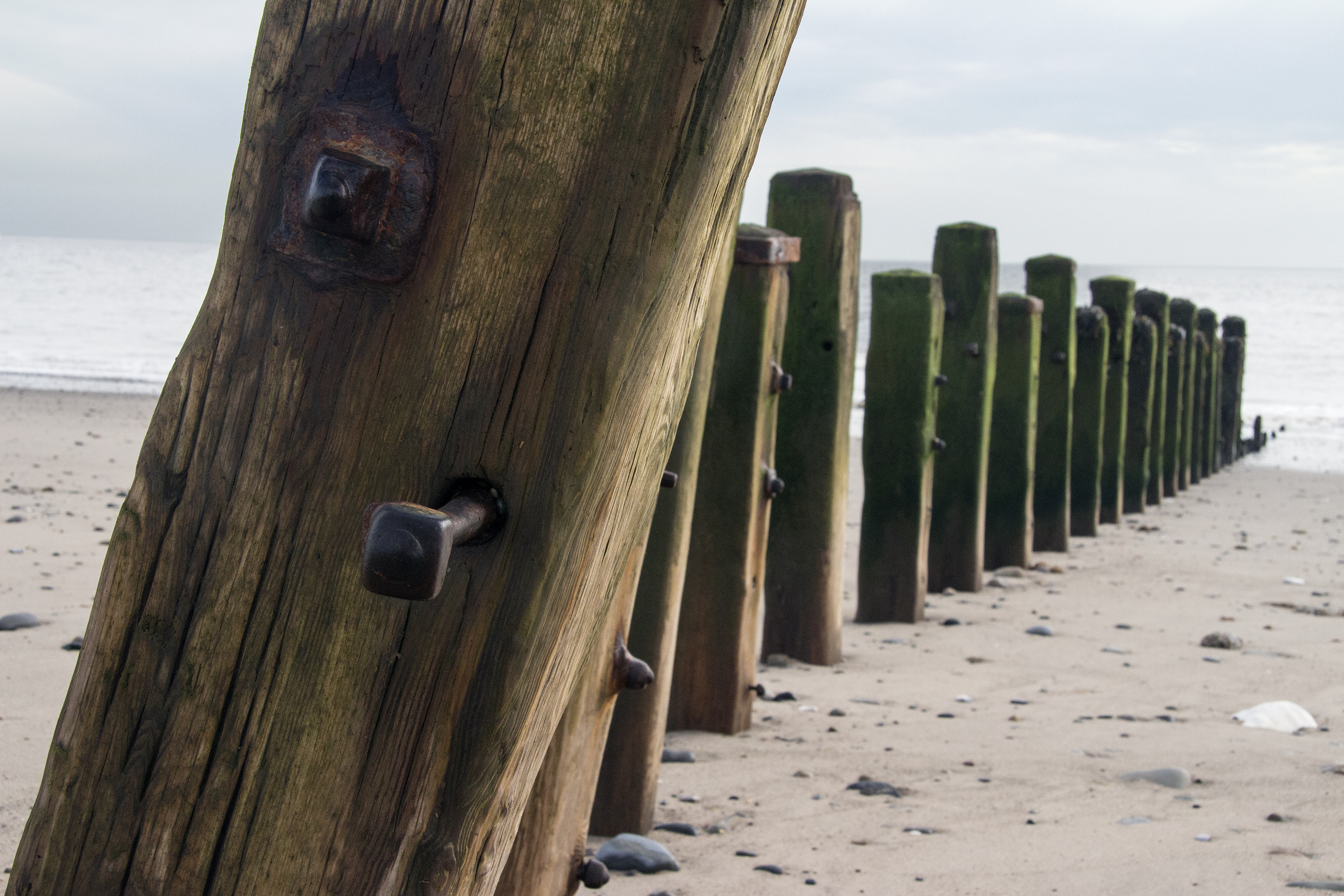The image captures a desolate beach scene dominated by a series of old, weathered wooden poles, which were likely the supports of a dismantled pier or a surf break barrier. The beach itself is a mix of sand, rocks, and shells, creating a rough terrain. In the foreground, one of the wooden supports is tilted about 30 degrees to the right, appearing to struggle against the forces of nature. These dark, brown stumps, about 20 to 30 in number, stretch into the distance, progressively showing more green hues as they recede towards the horizon. Many of these supports are studded with thick, rusty nails and large metal bolts, remnants from their original construction. The scene is framed by a cloudy sky, suggesting a potential storm, giving the image an ominous yet captivating atmosphere. The ocean water is visible primarily on the left and right sides of the photo, with the middle ground dominated by the line of poles leading towards where the water meets the sky. The entire image evokes a sense of erosion and abandonment, a testament to the relentless passage of time and tides.